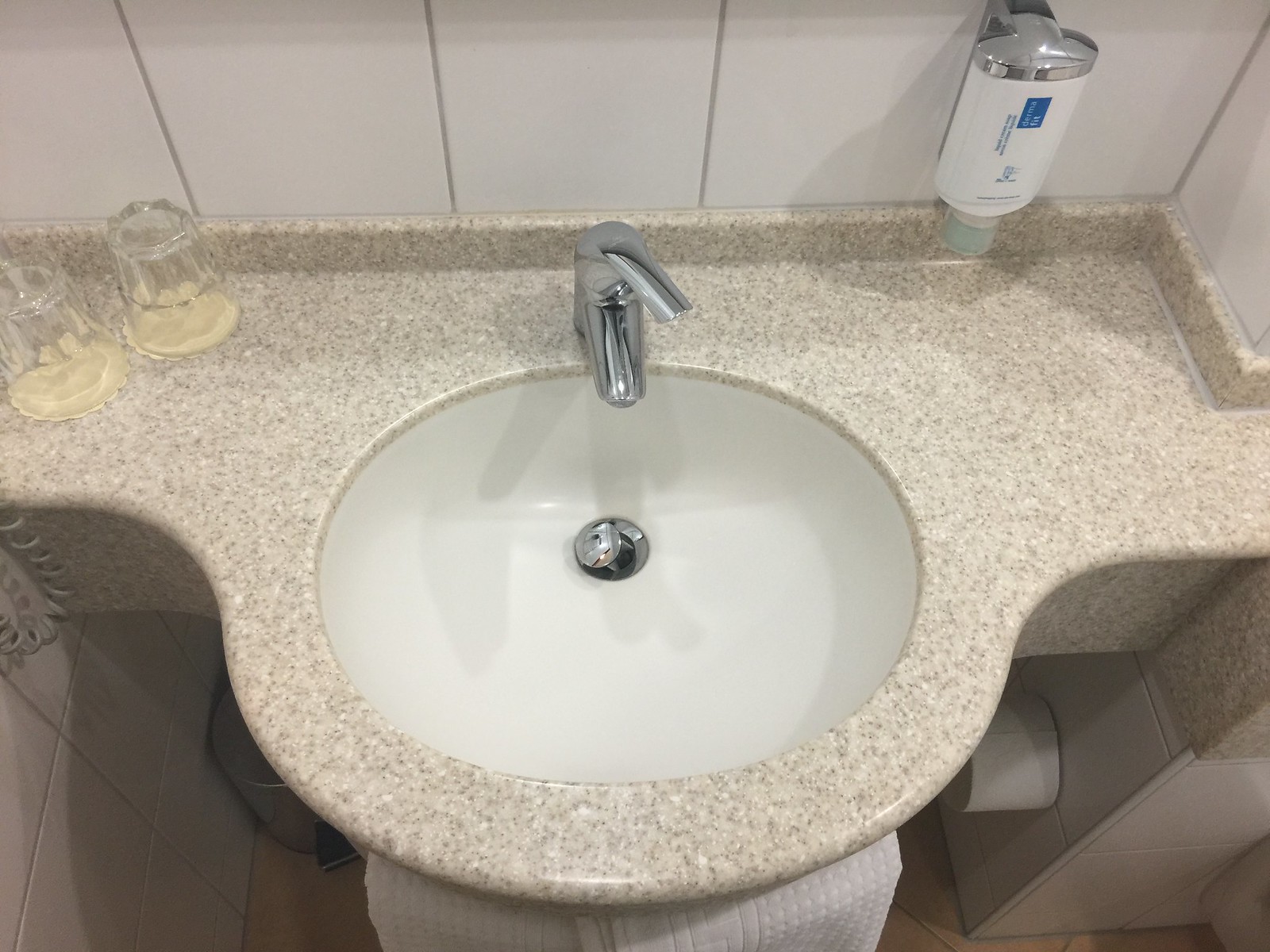This photograph captures a modern bathroom sink and counter, likely situated in a hotel, featuring a detailed array of amenities. The countertop is composed of a marble-inspired composite material in shades of gray and beige, accented with white specks. It extends around a white porcelain sink basin. A single chrome faucet, equipped with a lift mechanism for water activation and temperature control, occupies the sink's rear. To the left, the sink’s drain plug dangles slightly, adding a casual touch to the scene.

On the counter, two clear glass cups, inverted on cream-colored doilies, are positioned to the left. A bottle of liquid soap or possibly shampoo also lies inverted. The backdrop includes a large white tile backsplash, reinforcing the bathroom's clean, minimalistic design. Below the counter, white hand towels hang neatly in front, while a roll of toilet paper and coiled telephone cord are tucked off to the left, alluding to the possibility of this space being in a hotel. This meticulously arranged setting indicates a fresh, welcoming environment.